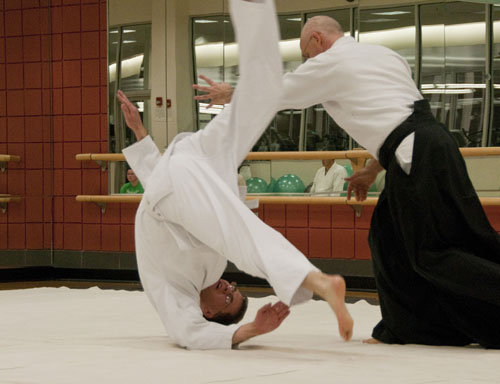This vintage-style action photograph captures an intense martial arts event featuring two men in the midst of a dynamic move. The man on the right, dressed in a white shirt and black billowing pants with a black belt, extends his hand towards the man on the left, who appears to be in the process of flipping or having just been struck. The man in white, both his shirt and pants, is visibly airborne and upside down, his head almost touching the white mat below. His legs are in motion, with one nearly reaching the ground while the other is elevated; his left hand is poised defensively in the air behind him, and his right arm is curled beneath his legs. This dramatic moment unfolds in a room with an Asian-inspired brown wall, bars encasing reflective mirrors, and a wall of windows. The scene is further energized by the presence of an audience in the background, some holding green balloons. The man in white seems surprised, his glasses emphasizing his expression.